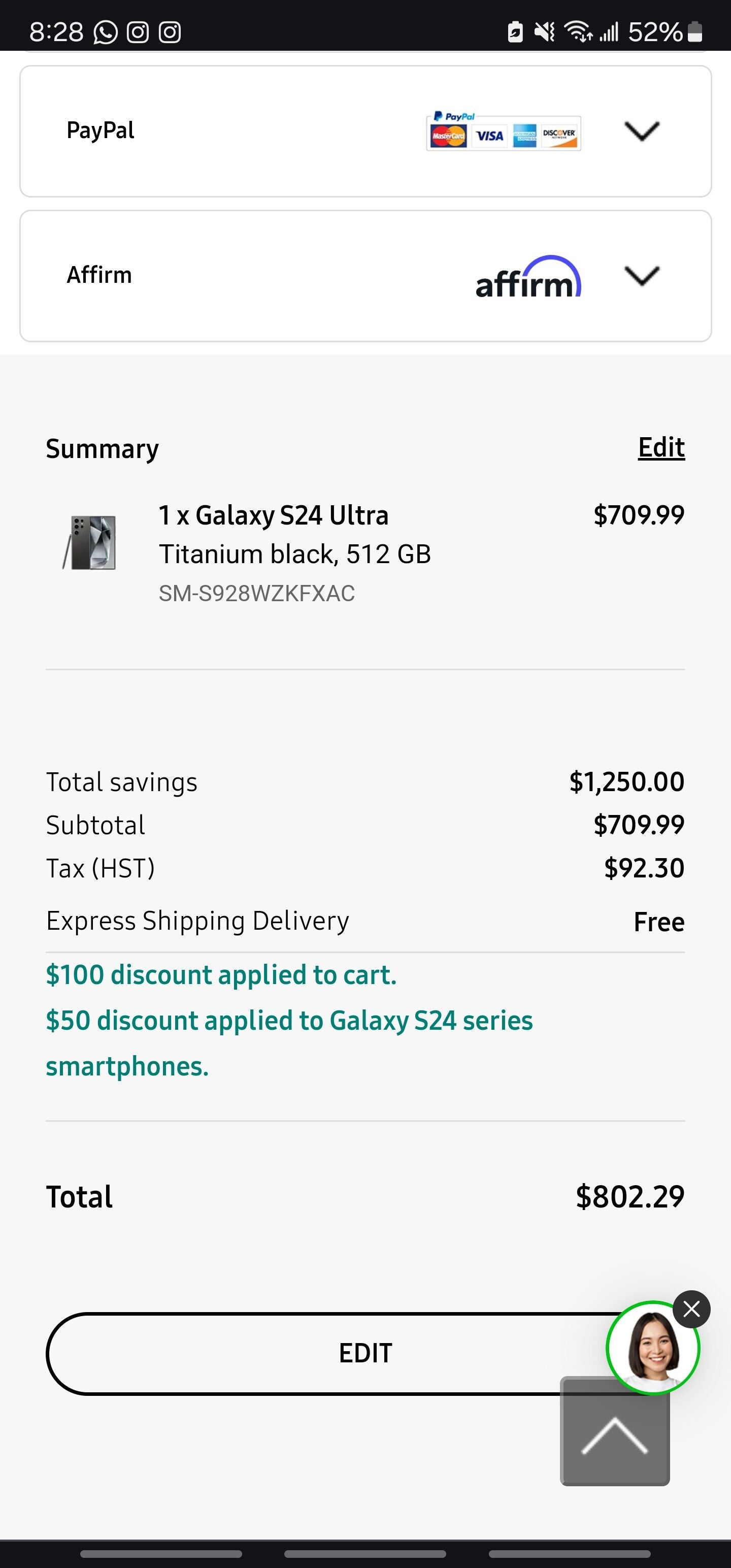A mobile phone screenshot captures the user's attempt to purchase a Samsung Galaxy S24 Ultra in Titanium Black with 512GB storage. At the top left, the screen shows the current time as 8:28, alongside icons representing open applications. The top right corner displays critical phone indicators, including a battery level at 52%, cell service signal, Wi-Fi connectivity, and other status icons. 

The page prominently offers several payment methods, such as PayPal, Visa, MasterCard, American Express, and Discover, with an additional option for Affirm payment plans. The item details show one unit of the Samsung Galaxy S24 Ultra priced at $709.99. Detailed savings information highlights a significant discount of $1,250, bringing the subtotal to $709. 

Additional costs include a tax of $92.30, but express shipping is free. Applied discounts are also noted. The final total for the purchase is calculated at $802.29. An "Edit" button is visible at the bottom of the screen, suggesting the option to modify the order.